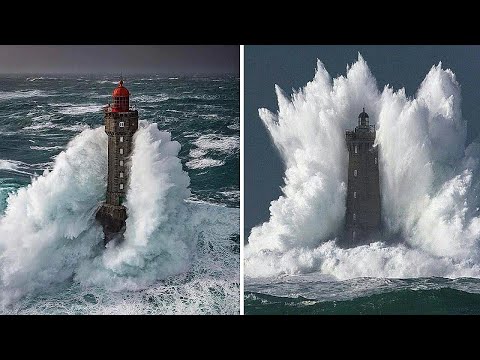This image, likely a still taken from a video, features a rectangular frame wider than it is tall, with black bars on the top and bottom and divided in the middle by a white line, creating two distinct photographs. 

On the left side, a brown lighthouse with a red top stands resolutely in the ocean, surrounded by choppy green waters. A massive wave, frothy with white water, surges dramatically around the structure, almost enveloping it in a watery embrace. The sky above is dark gray, and the whole scene gives an impression of nature's raw power against the steadfast lighthouse.

On the right side, another lighthouse with a dark gray top is similarly besieged by tumultuous waters. The ocean here is also green and treacherous, with violent white waves crashing around the lighthouse, even rising past its summit. The darker bluish-gray sky serves as a foreboding backdrop, amplifying the dramatic moment captured.

Both images convey an intense atmosphere of stormy seas against tall, resilient lighthouses guiding ships through the tempest.